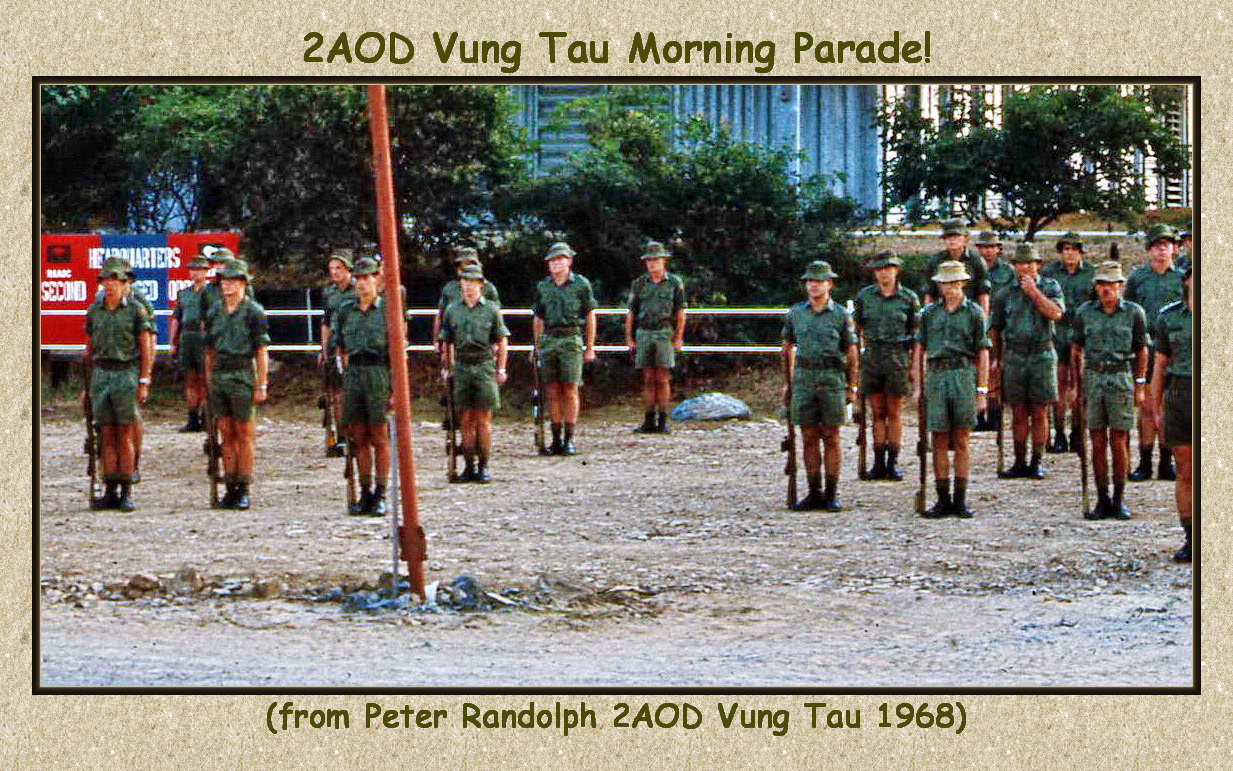The image is a rectangular photograph set within a grayish-beige border, framed by a black outline. It depicts an outdoor military scene featuring Asian soldiers standing at attention on sandy, rocky ground. These soldiers, wearing green short-sleeved shirts, green shorts, and black combat boots, are lined up with rifles pointed down at their right sides. They have hats on, some khaki, and some army green. In front of them stands a large orange pole embedded in the ground. In the background, there are buildings, trees, and a scoreboard on the left. The caption at the top of the image reads "2AOD Vung Tau Morning Parade!" in green, and the bottom text within the border states, "From Peter Randolph to AOD Vung Tau 1968."